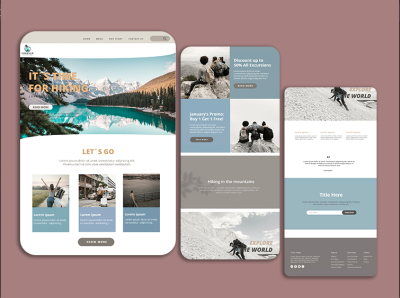The image showcases a muted peachy brown background upon which there are representations of a tablet and two cell phone screens, though the low resolution renders many details indistinct. On the tablet screen, a tan strip runs across the top, featuring navigation indicators for four sections. However, the text is too blurred to read.

In the top right corner of the tablet screen, there is a search bar. Below this lies a white strip; on the left side of this strip, a logo is visible. Beneath the logo is a photograph depicting a serene mountain pond or lake, surrounded by snow-capped peaks and green conifer trees. Overlaid on the image, in tan-colored text, it reads "It's time for hiking." Below this, the phrase "Let’s go" is visible, but any further text in black is illegible.

Below the main photograph, there are three vertically aligned images in a row, but the content within these is unclear. Further down, there's a gray button with white text, which is also unreadable.

To the right of the tablet screen, there is a smaller, thinner rectangle resembling a cell phone screen. In its top left corner is a photograph, and in the top right corner, there is a blue square, likely a button, the details of which remain indistinct.